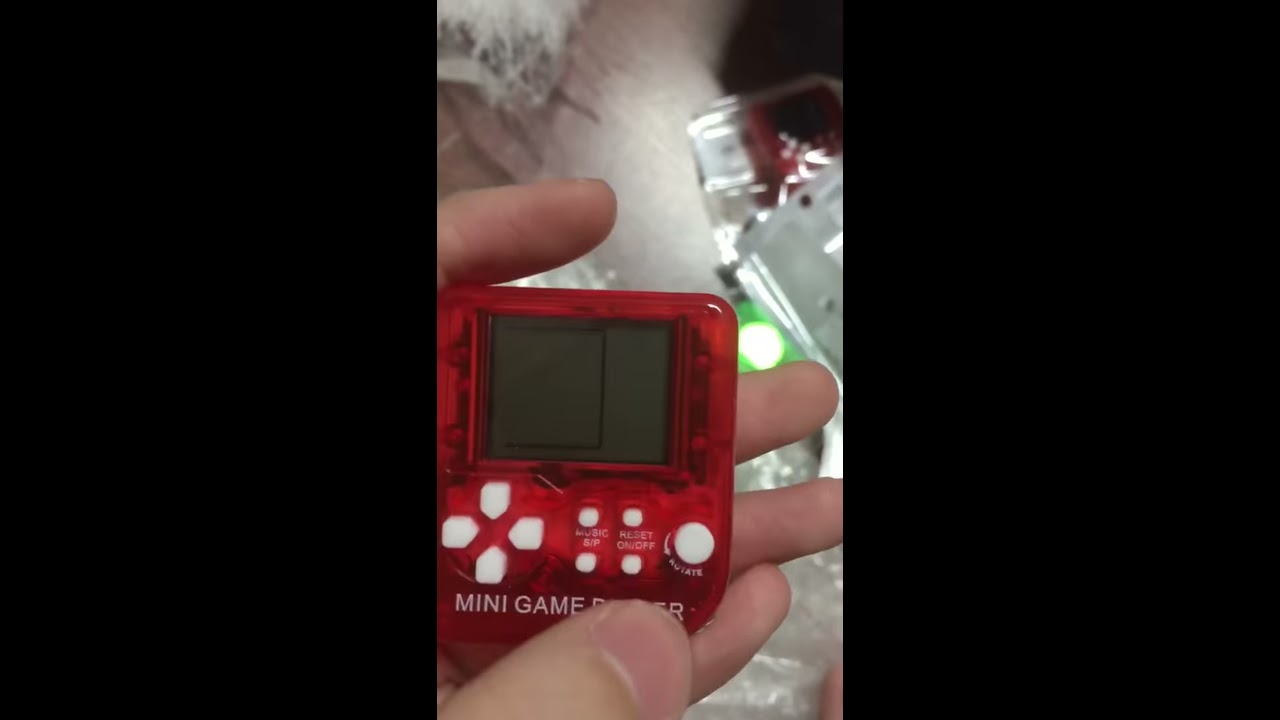This close-up photo, framed by two black rectangles on either side, vividly captures a person's hand holding a small, retro-style, red video game device. The device prominently displays the text "mini game player" in white, partially obscured by the person's thumb. The person's hand is oriented with the thumb facing downward and the fingernails visible, while the palm faces upward. The device features four white buttons aligned on the left side and two additional rows of smaller buttons labeled with functionalities such as "music up" and "reset/on/off." A larger button is situated to the right of these controls. The screen of the device shows an incomplete rectangle, reminiscent of basic, old-fashioned digital graphics. The photo's setting includes what appears to be a bedroom environment with a lace-trimmed pillowcase and a shiny bed cover visible in the background, alongside other indiscernible items. Additionally, the background features bright, shiny decorations, possibly indicating a festive, holiday ambiance.